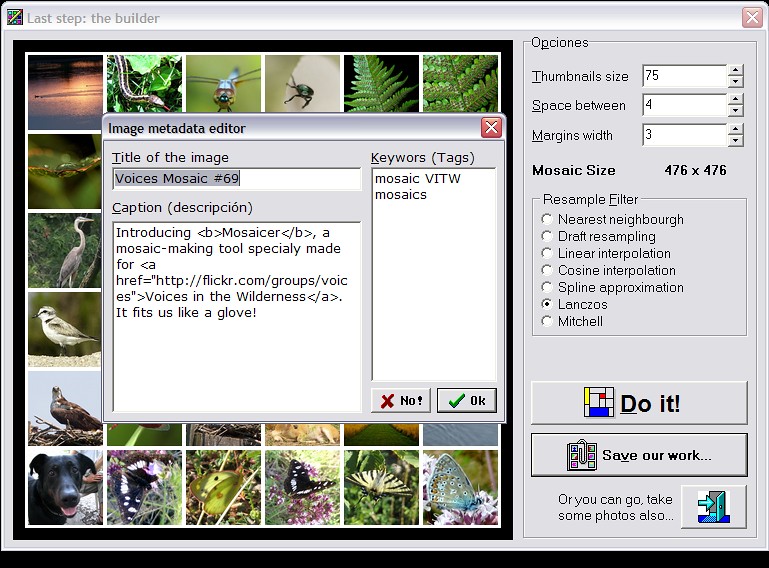The image depicts a screenshot of an old-fashioned Windows computer interface displaying a mosaic editing tool. At the top, the text reads "Last Step, The Builder." A central pop-up window, titled "Image Metadata Editor," shows details such as "Voices Mosaic Number 69" and a caption introducing "Bee Mosaica," designed for the Flickr group "Voices in the Wilderness." Surrounding the pop-up, thumbnails of diverse animals and nature, including dogs, birds, a snake, insects, fish, plants, and butterflies, are arranged in a grid pattern. These thumbnails feature vibrant colors like green, black, yellow, blue, red, purple, brown, and gray, somewhat obscured by the pop-up. To the right of the screen, editing options such as "Thumbnail Size," "Space Between Margins," "Begin Mosaic Size 476 by 476," and various resampling techniques are listed. Below these, buttons labeled "Do It," "Save Our Work," and "You Can Go Take Photos Elsewhere" provide user interaction options. The scene captures the tool's interface, giving a detailed look at both the editing options and the colorful array of images being used to create the mosaic.